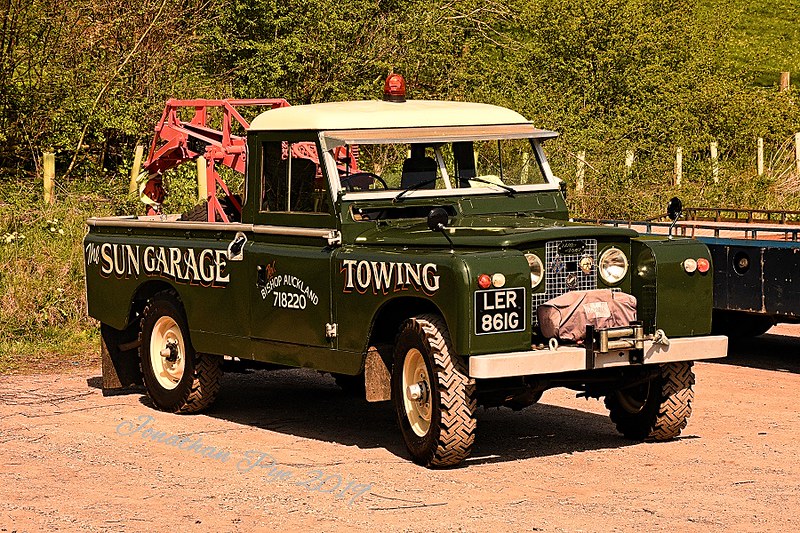The image features a vintage green tow truck that appears to have originated from a Willys Jeep, with a characteristic front end design and headlights set towards the center of the hood. It's modified into a pickup truck configuration without a back, equipped with hefty snow or mud tires, a winch mounted on the front bumper, and a crane lift arm at the rear. The tow truck has an off-white top and a small yellow alert light on the cabin. On its side, it is branded with the text "Sun Garage Towing" and the location "Bishop, Auckland, 718220". The license plate reads "LER861G". The truck is parked in an area surrounded by many trees, and inside the back, there seems to be a reddish object. The surroundings and the classic design emphasize its rustic and utilitarian charm.